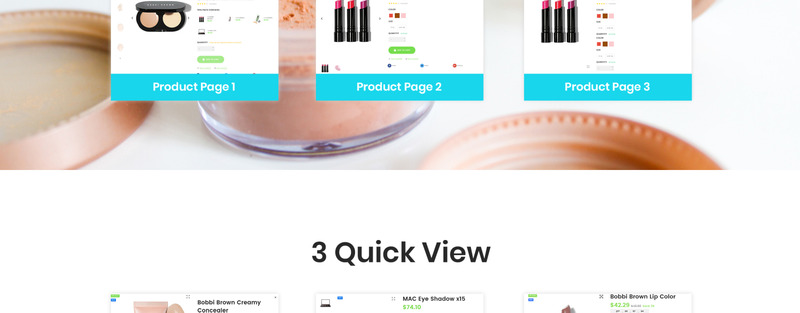This image is a detailed screenshot of a website. The URL is not visible in the capture. The upper half features a background image, likely showcasing a tan-colored makeup product. Positioned in front of this backdrop are three square boxes, each representing a different product page labeled "Product Page 1," "Product Page 2," and "Product Page 3" against a blue rectangle at the bottom of each square. The product in the first square appears to be a makeup item housed in a circular container, seemingly consisting of two compartments or items inside. The second and third squares each display three lipsticks, though the text details are too small to read. 

The lower half of the screenshot contrasts with a white background and prominently displays the title "3 Quick View." Below this title are three additional boxes that are partially cut off. Despite the truncation, partial text can be seen, identifying one product as a concealer, another as MAC eyeshadow, and the third as a brown lip color. The majority of the details in this portion of the image are obscured.